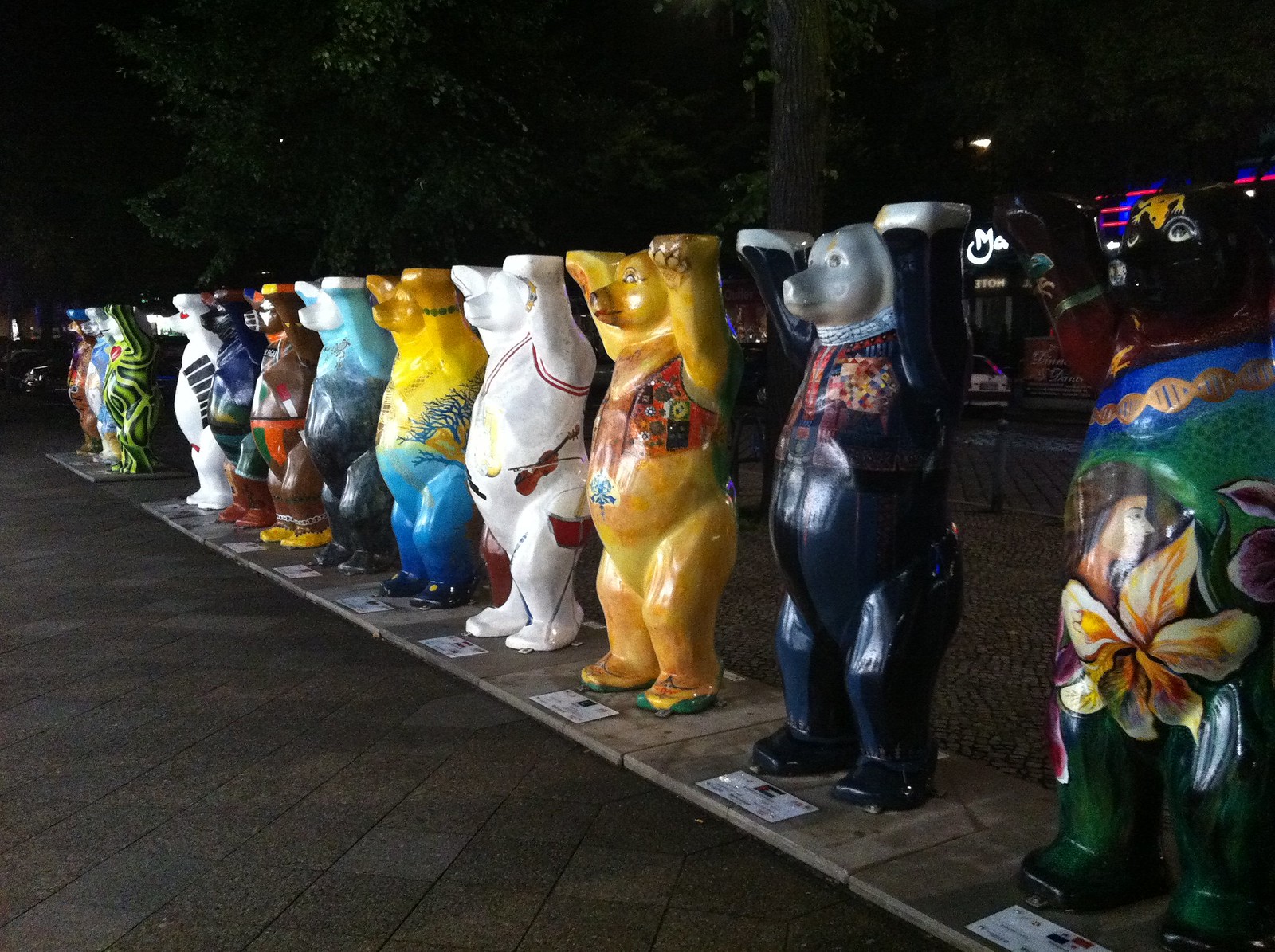This nighttime photograph captures an art installation of twelve life-sized fiberglass bear statues, each uniquely and elaborately painted by different artists. The bears are arranged in a horizontal line, starting from the upper left corner and stretching to the lower right. All the bears stand on gray cement tile slabs with labels in front of them, though the text on the labels is not legible.

Each bear is poised upright on its hind legs with its front paws raised above its head as if holding something. The variety in their coloration and design is striking:

1. **First bear:** Black head, green legs, with a detailed painting of a woman and a flower on its midsection.
2. **Second bear:** Appears to wear a navy blue and black suit on a white body.
3. **Third bear:** Yellow with a colorful vest.
4. **Fourth bear:** White with red musical instruments, including a violin and a drum, painted across its body.
5. **Fifth bear:** Blue bottom, yellow top, decorated with blue trees.
6. **Sixth bear:** Dark blue bottom, seafoam green top, details indistinct.
7. **Seventh bear:** Predominantly brown with various color designs.
8. **Eighth bear:** Green bottom, blue top, designs indistinct.
9. **Ninth bear:** White with black keyboard imagery painted on it.
10. **Tenth bear:** A swirl of various green hues.
11. **Eleventh bear:** Details unclear.
12. **Twelfth bear:** Details unclear.

In the background, fluorescent and neon lights suggest a busy area, contributing to the vibrant atmosphere. Green leaves and a tree are visible, adding a natural element to the setting. The combination of detailed artistry on each bear and the illuminated, bustling environment creates a captivating visual display.